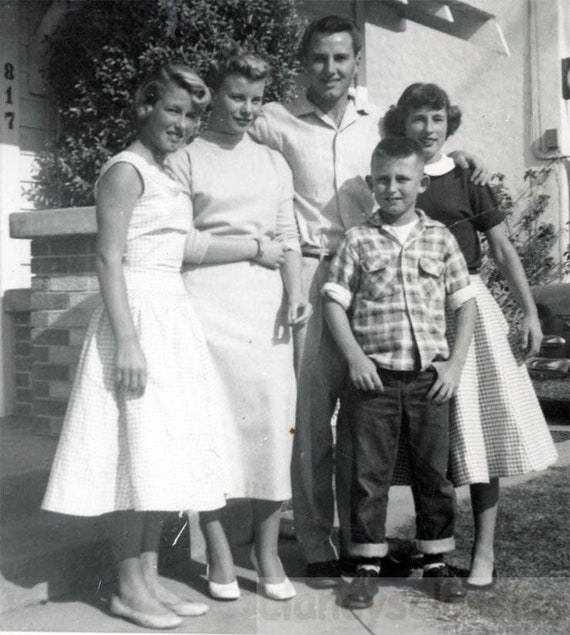This black and white photograph, likely from the 1950s, captures a family of five arranged in front of a house with the number 817 visible above the entrance. The man, tall and clean-shaven, stands confidently in light-colored pants and a light-colored shirt, which underline the era's fashion. To his side is a young lady in a beige dress, identifiable by her short blonde hair and white heels. Another lady stands beside her in a light-colored checkered dress, also with short hair but distinguished by her sleeveless gown and white pump shoes. On the other side of the man, there's a young girl in a dark top with a plaid skirt, her hair styled with bangs and curls on the sides, embodying youthful innocence. At the front stands a young boy, likely around eight or nine years old, dressed in blue jeans with rolled cuffs, a plaid shirt over a white undershirt, and black Oxford shoes. The background hints at a family's pride in their home, with visible steps, brickwork, and hints of floral and plant life, all bathed in sunlight. The family's unified gaze and smiles towards the camera evoke a sense of warmth and togetherness from a bygone era.